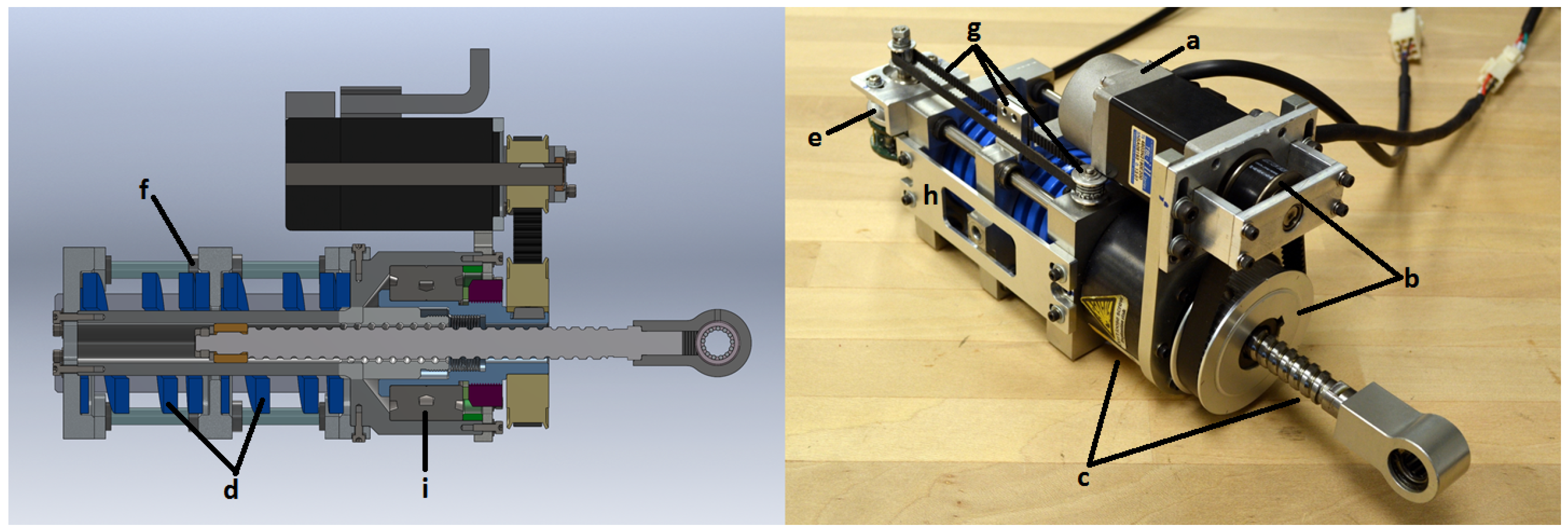This rectangular image, approximately six inches wide and two inches high, is divided into two distinct sections: the right side features a real-life photograph of a mechanical device, while the left side presents a detailed computerized rendering of the same device against a grayish background. The device is positioned on a light brown wooden floor in the photograph, providing a realistic context. 

The mechanical device appears intricate and multifunctional with several key components. At the forefront, it has a small ratchet end attached to a blue spring-like core, leading to a spiral metal piece that can extend in and out. Adjacent to this is a golden-colored cylinder and a knob that connects to a screw cable or bolt running through the core. Behind these features, there is a motor accompanied by driving belts at the top. Several black electrical cords emerge from the upper right section of the device, equipped with connectors.

The rendering on the left side of the image meticulously labels various parts of the device with letters such as A, B, C, E, G, H, F, D, and I, using lines to point to each corresponding section. The detailed markings in the diagram highlight the functional aspects and connectivity of the device, suggesting it as an electrical component capable of generating power.